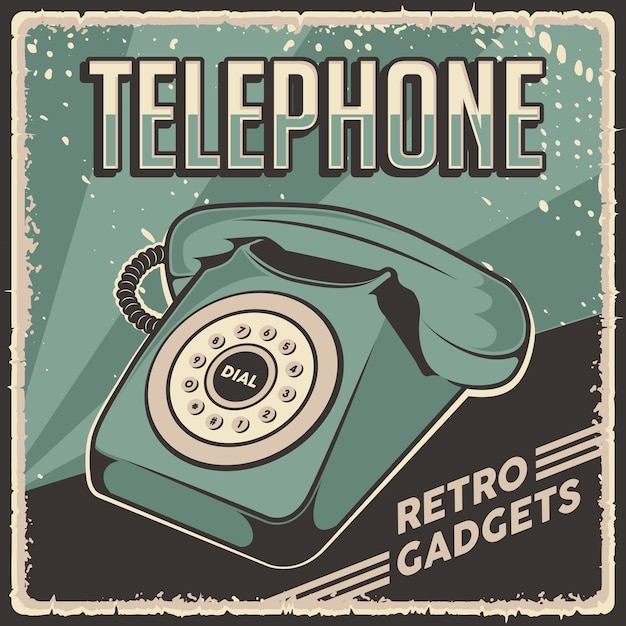In this digitally created, retro-styled advertisement, the word "TELEPHONE" dominates the upper center of the image in bold, two-tone block letters – the top half white and the bottom half a vintage teal blue. Set against a teal blue background with the lower third transitioning into black diagonally, this old-fashioned image showcases a classic rotary dial telephone beneath the bold text. The telephone, matching the teal blue color scheme, features a circular dial with numbers from 0 to 9, along with a star (*) and pound (#) symbol. The word "DIAL" is embedded in the center of the circle. The image exudes a deliberately worn, vintage aesthetic with discolored, faded tan and light brown edges leading into a darker black border. In the lower right corner, white text against the black background reads "Retro Gadgets," accompanied by three horizontal stripes above and below the text, enhancing the nostalgic feel.